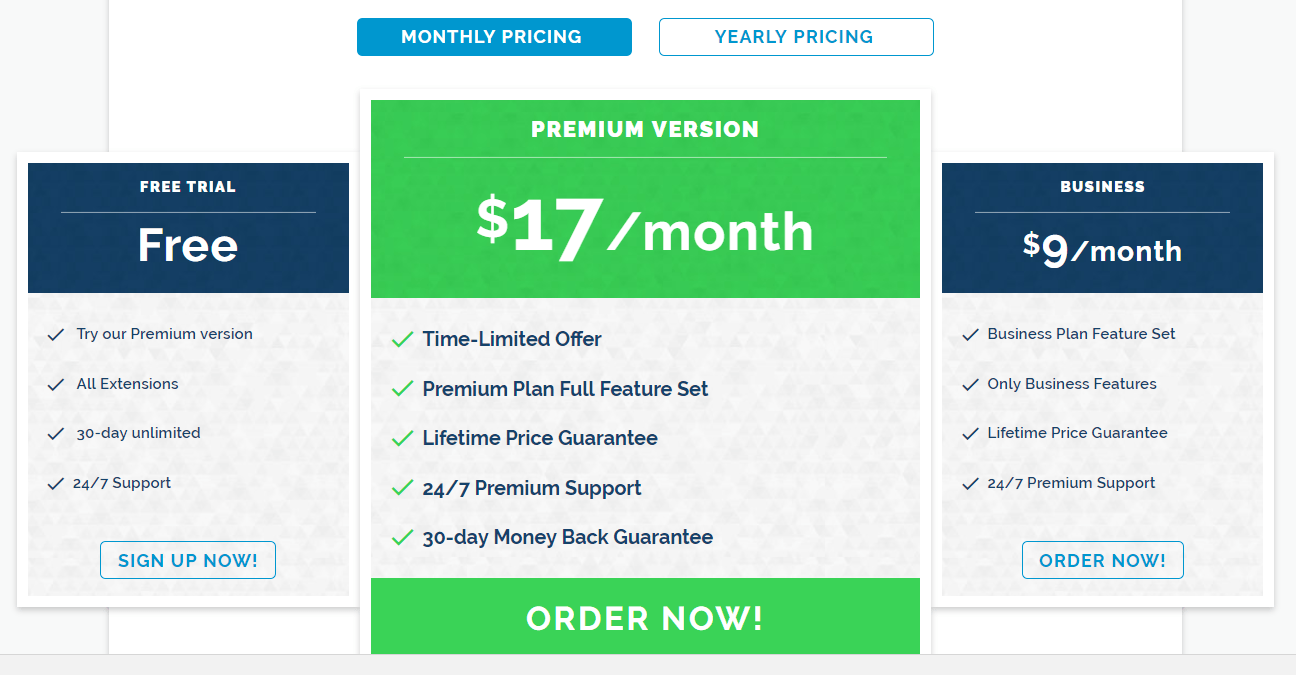This screenshot displays a comparison between monthly and yearly pricing plans, emphasizing the currently selected monthly pricing option, highlighted in a dark blue box. There are three distinct subscription options available:

1. **Free Trial:**
   - Label: Free
   - Details: "Try our premium version, all extensions, 30-day unlimited, 24-7 support"
   - Button: Blue "Sign Up Now"

2. **Premium Version:**
   - Monthly Cost: $17
   - Offer: Time-limited offer
   - Features: Full feature access, lifetime price guarantee, 24-7 premium support, 30-day money-back guarantee
   - Button: Blue "Order Now"
   - Highlight: Displayed within a green box to draw attention

3. **Business Plan:**
   - Monthly Cost: $9
   - Features: Business plan feature set, lifetime price guarantee, 24-7 premium support
   - Button: Blue "Order Now"
   - Highlight: Displayed within a navy blue box

Overall, this detailed pricing comparison aims to help users choose between free, premium, and business subscription plans with clear indicators for pricing and support features.